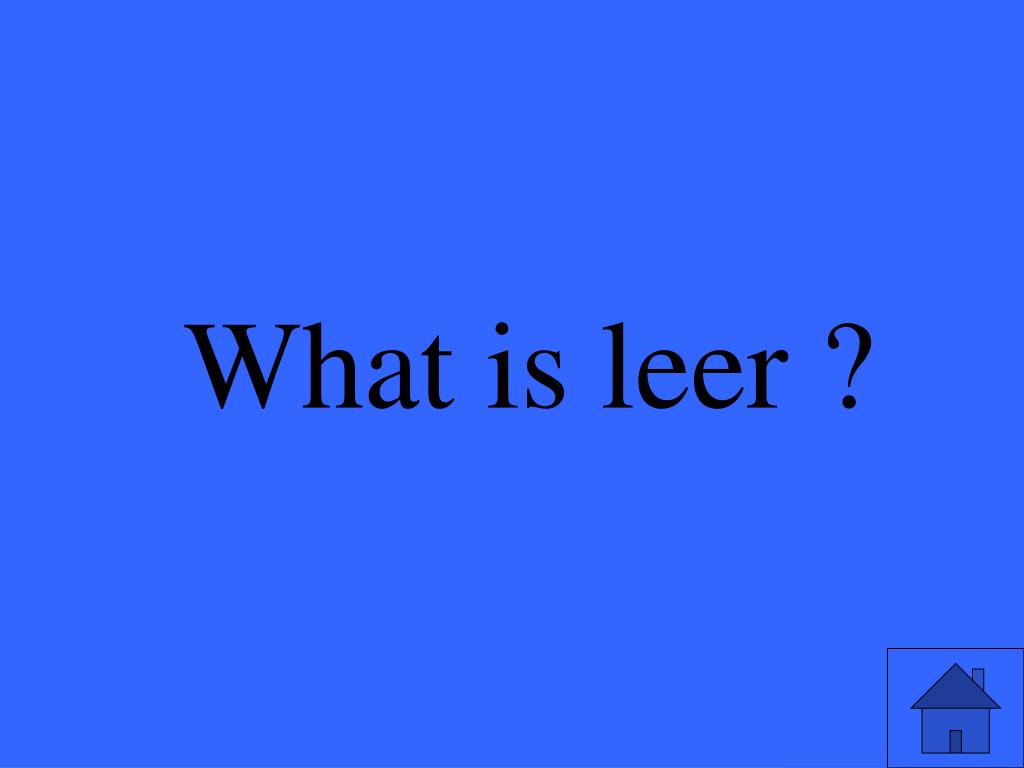The image depicts a slide or presentation with a solid deep blue background. At the center of the slide, the text "What is Lear?" is displayed in black Arial font, stretching across the width of the image. In the bottom right corner, there is a simple sketch of a house, characterized by a small door, a triangular roof, and a chimney protruding from the right side of the roof. The overall design and style suggest a PowerPoint presentation, with the primary colors being blue, black, and gray.